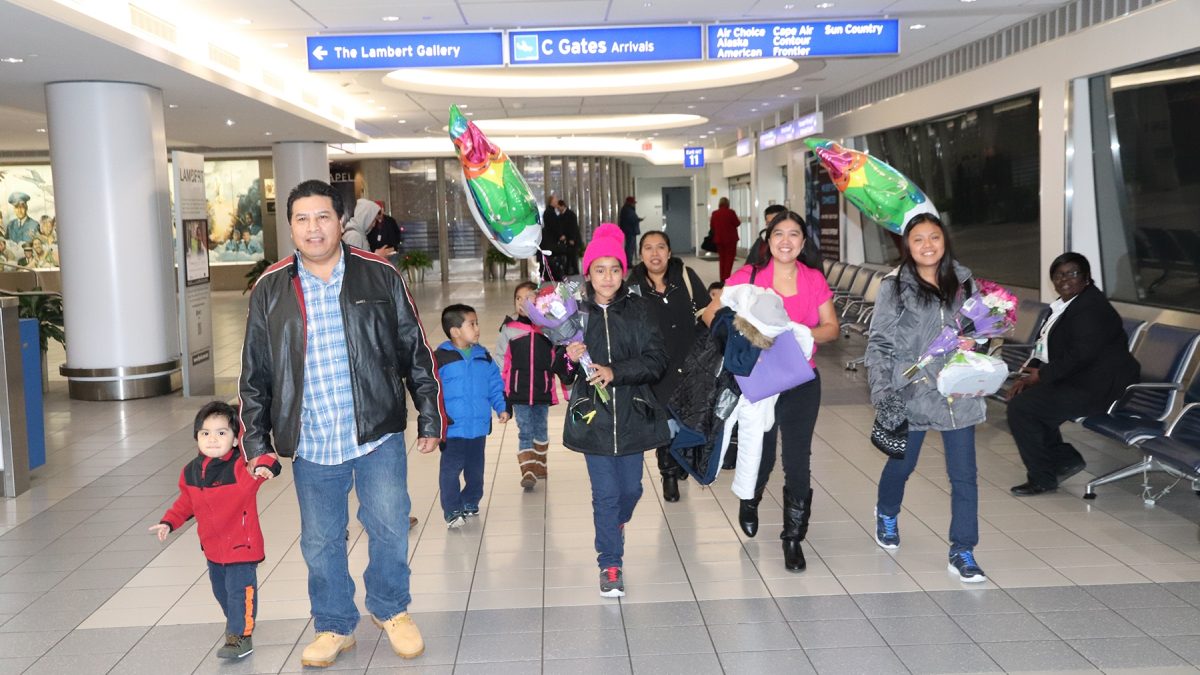In this detailed photograph, a family of eight is walking through an airport terminal, heading toward the photographer. Centered in the image, the family consists of several females and a few males, all dressed in winter attire. A man in a black leather jacket can be seen toward the left, holding the hand of a young boy in a striking red jacket with black accents around the collar. The airport floor features a mix of white and gray tiles, providing a neutral backdrop.

On the upper left of the image are large circular white support columns, contributing to the spacious feel of the terminal. Above the family, various signs are visible. A prominent blue sign reads "The Lambert Gallery" with an arrow pointing left. Adjacent to it, a green sign states "Seagate's Arrivals," accompanied by an airplane symbol, and lists several airlines including Air Choice, Alaska, American, Cape Air, Contour, Frontier, and Sun Country. A partially visible sign displays the number 11 and other indistinct information.

To the left, large windows reveal the nighttime outside, and a row of blue chairs with silver handles lines the area. One chair is occupied by a woman with black hair, wearing a black long-sleeve shirt over a white shirt. Among the scattered travelers, a couple of family members are notably carrying bouquets and balloons, adding a festive touch to the scene. Despite the minimal overall crowd, the photograph captures a moment of arrival and familial camaraderie.